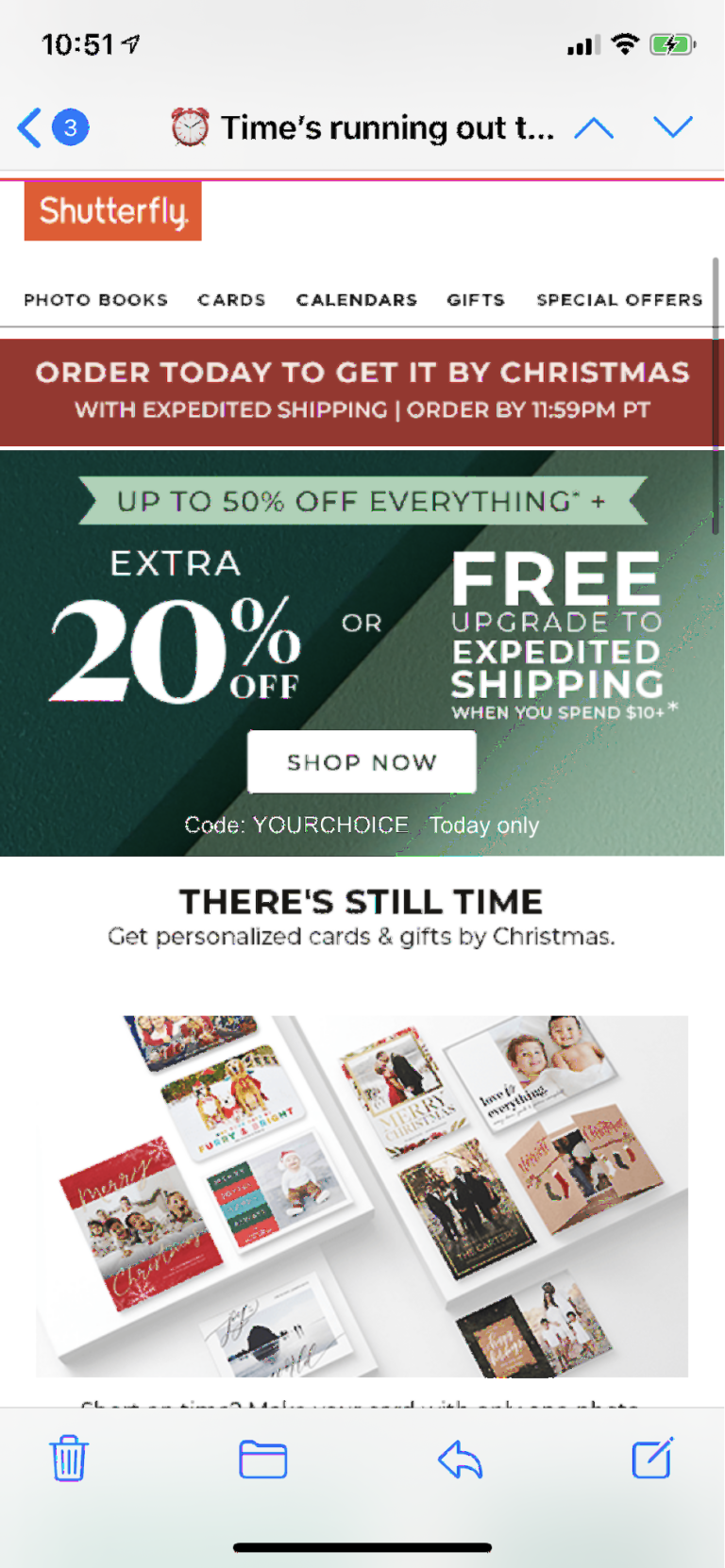This is a detailed and cleaned-up caption for the described image:

---

Screenshot of a smartphone-accessed website. The image is long and narrow. The top of the screen displays the time (10:51) alongside a small arrow. Connectivity indicators show three out of four signal bars, a Wi-Fi signal, and a charging battery icon.

Below, a navigational bar includes a left-facing arrow and a blue circle marked with the number three. Next to them, an alarm clock icon appears with a partially visible text implying "time's running out." Up and down arrows likely represent scroll controls.

The website headline reads "Shutterfly," followed by clickable links for "Photo Books," "Cards," "Calendars," "Gifts," and "Special Offers." A banner message urges, "Order today to get it by Christmas with expedited shipping. Order by 11:59 p.m. Pacific Time."

The next section features a green two-toned diagonal split, darker green on the left and lighter green on the right. A promotional banner declares "Up to 50% off everything," accompanied by a plus sign. Below in the green area, additional offers are detailed: "Extra 20% off or free upgrade to expedited shipping when you spend $10+. A white box labeled "Shop Now" includes the code "Your Choice," indicating the promotion is valid for today only.

Further down, a highlighted message states, "There's still time, get personalized cards and gifts by Christmas," illustrated by a photo of various custom Christmas cards. These cards are created by users uploading their photos, which Shutterfly prints and mails back to them.

At the bottom of the screen, four icons are displayed: a trash can (delete), a folder (save), a left-facing arrow (back), and a symbol resembling a share function (a box with an ink pen or pencil).

---